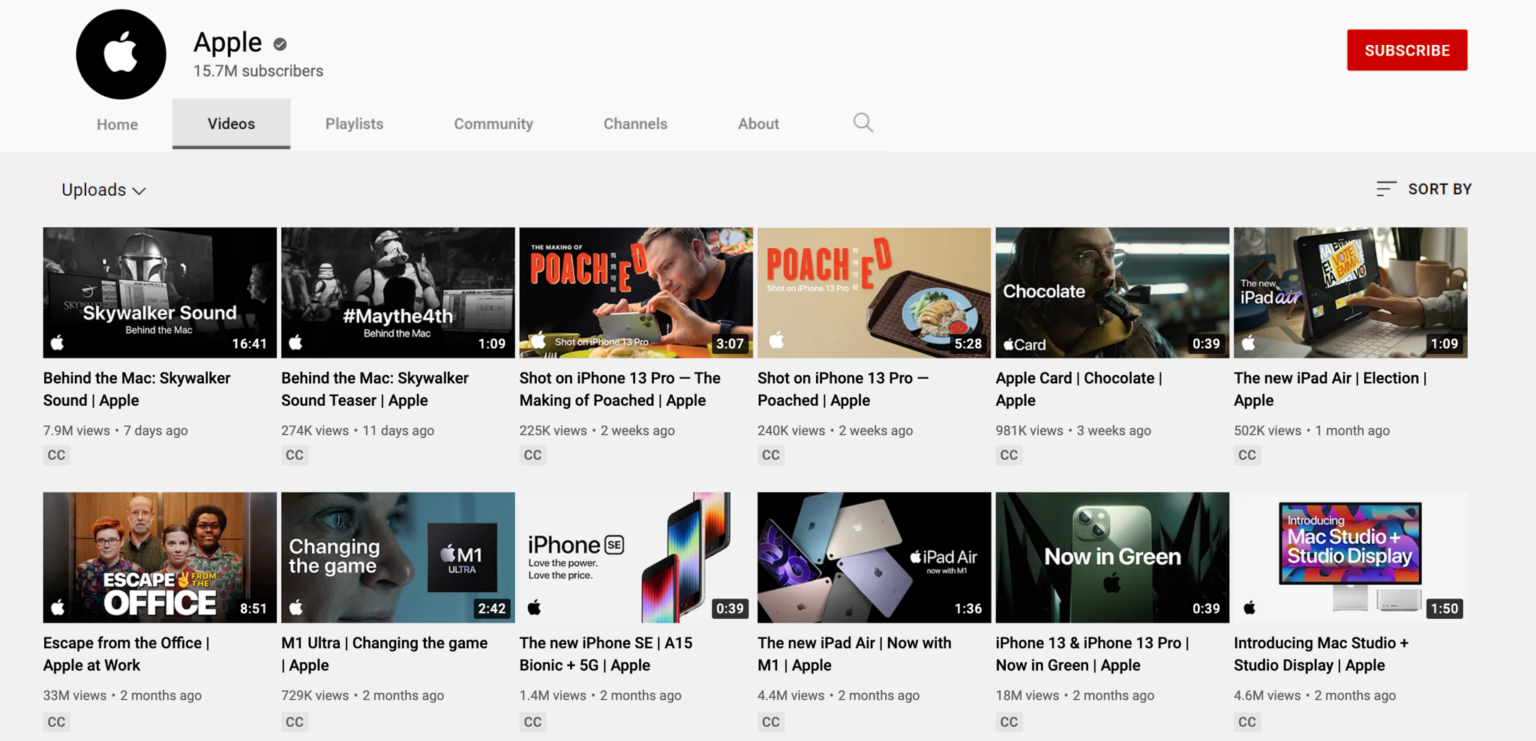The image is a screenshot of an Apple website with a light grey background. Positioned at the upper left corner is a black circular icon featuring the Apple logo, accompanied by the word "Apple" written beside it. Below this, it indicates that there are 15.3 million subscribers. 

At the upper right corner, a red "Subscribe" button is prominently displayed. Adjacent to it are navigational links labeled as "Home," "Videos," "Playlists," "Community," "Channels," and "About," with a search icon following these options. The "Videos" tab is currently selected.

Beneath this section, the "Uploads" header introduces a display of two rows containing five video thumbnails each. These thumbnails feature a mix of black and white as well as colored images.

- The first video on the left is titled "Behind the Mac: Skywalker Sound | Apple," followed by a teaser titled "Behind the Mac, Skywalker Sound Teaser | Apple."

- Continuing along the row, the next two videos are titled "Shot on iPhone 13 Pro | The Making of Poached | Apple" and "Shot on iPhone 13 Pro | Poached | Apple," respectively.

- Concluding the first row is a video titled "Apple Card: Chocolate | Apple."

The second row begins with "The New iPad Air: Election | Apple," followed by "Escape from the Office | Apple at Work."

- Next is a video titled "M1 Ultra: Changing the Game | Apple," then "The New iPhone SE | A15 Bionic + 5G | Apple."

- The final video in this row is titled "The New iPad Air: Now with M1 | Apple."

At the very bottom right of the screenshot is a thumbnail for a video titled "Introducing Mac Studio + Studio Display | Apple."